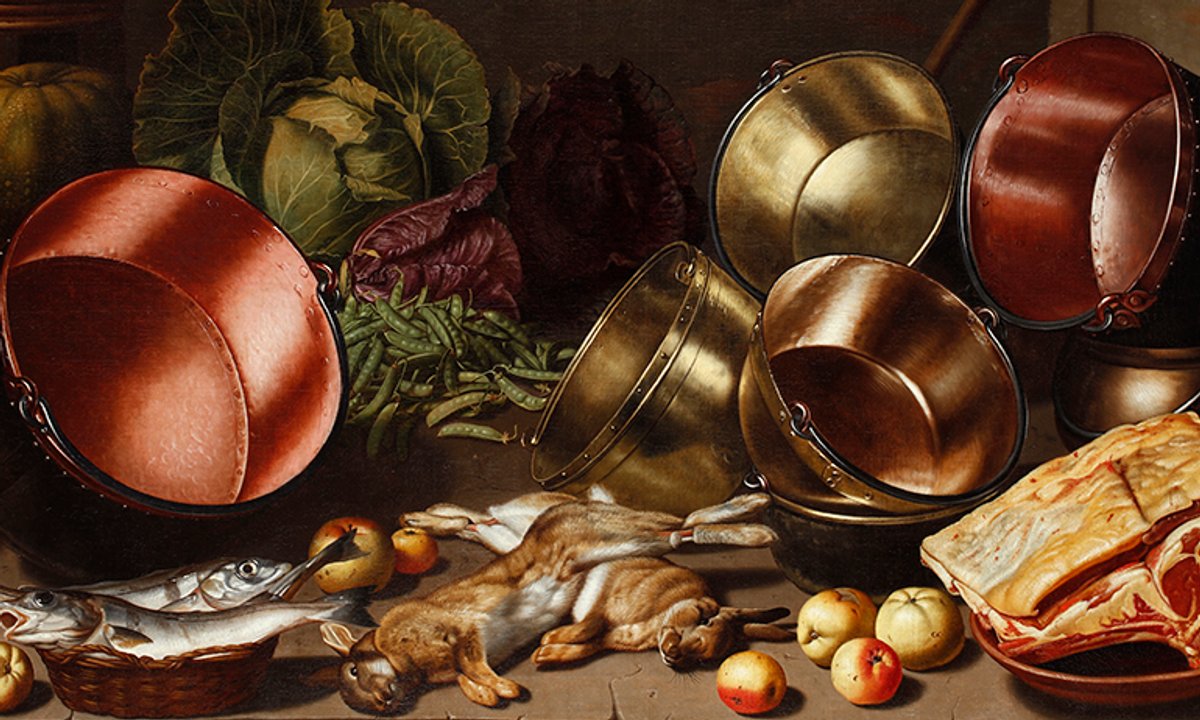This detailed painting of a historical kitchen scene is bursting with various elements that give a glimpse into meal preparation before the advent of grocery stores. On the right side of the painting, there are five brass pots, tilted at an angle that reveals their interiors. Among these pots are fresh vegetables, including a green cabbage, a red cabbage, and an arrangement of green beans. Moving to the left, a larger pot is positioned to display its copper lining. At the bottom left corner, there is a basket filled with freshly caught fish, adding to the authenticity of the scene. Next to the fish are a few scattered apples and peaches on the ground. To the bottom right, a bowl containing an unidentifiable piece of red meat is visible, further suggesting preparations for a meal. Two dead rabbits lie cross-folded over one another, indicating they are next in line for skinning and cooking. The background is decorated with more vegetables such as lettuce and pinkish rhubarb, intricate details that reinforce the kitchen activity. This painting richly captures the essence of a bygone era's kitchen, readying for a sumptuous feast.